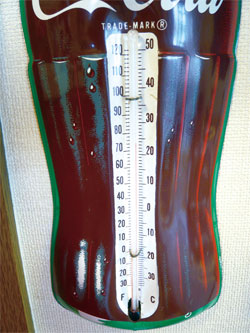This image features a vintage-style thermometer encased within a decorative Coca-Cola bottle, which is dark-colored to resemble real glass. The thermometer is set against a white background, with black numbers indicating temperature; Fahrenheit on the left side and Celsius on the right. The thermometer's backdrop is also white, providing a crisp contrast. In the photo's lower-left corner, a glimpse of wood grain suggests the surface it rests upon could be a table or wall. Supporting this, there's a white object beneath the thermometer with a textured surface and a green border, adding further context to its setting. The upper part of the Coca-Cola bottle decoration reveals part of the iconic logo, displaying the "Cola" in the recognizable font.